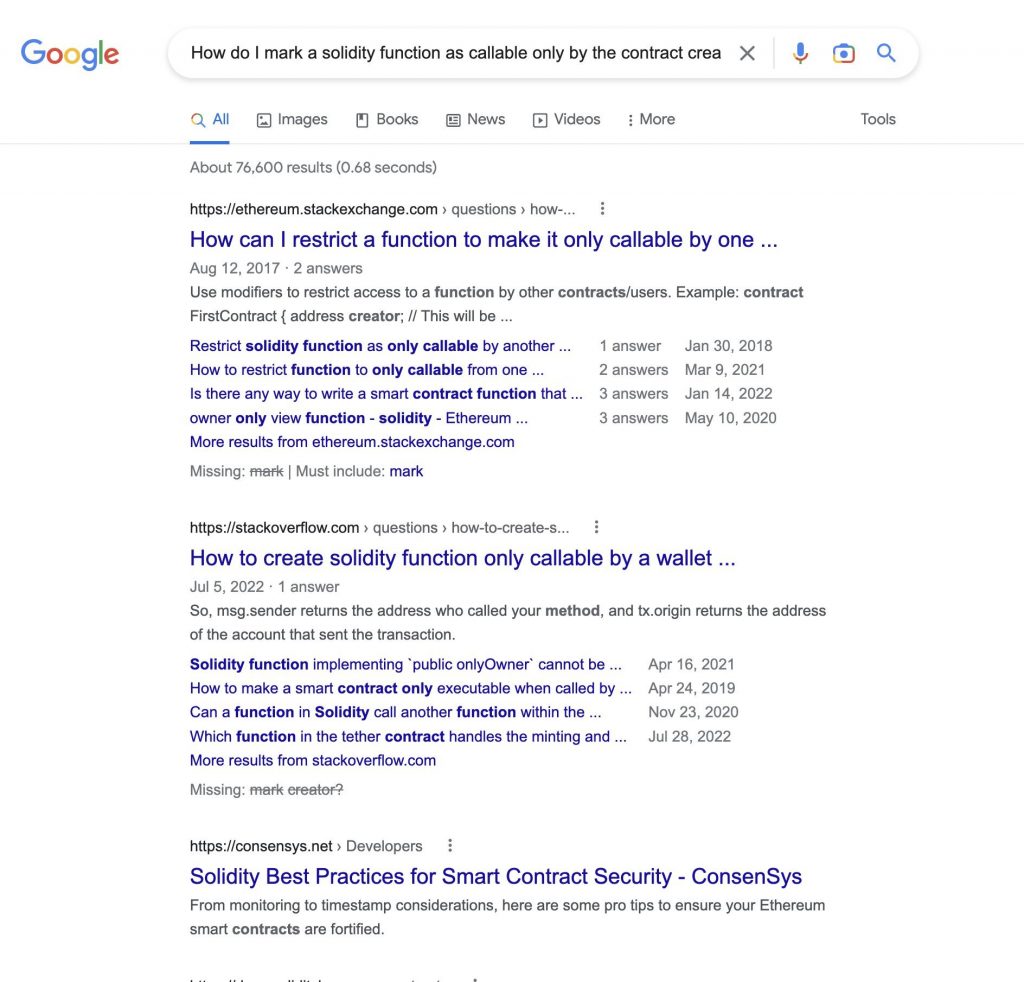This is a detailed caption that provides an in-depth description of the screenshot:

---

This screenshot captures a Google search page displaying results for the query, "how do I mark a Solidity function as callable only by the contract creator." In the top left corner, the iconic Google logo is prominently visible, followed by the search bar containing the query text. Below the search bar, the "All" tab is selected among the various options including Images, Books, News, Videos, More, and Tools.

Google has returned approximately 26,600 results in 0.68 seconds. The top result is from Ethereum.StackExchange.com, titled "How can I restrict a function to make it only callable by one ...", dated August 12, 2017, and features two answers. The snippet highlights the use of modifiers to restrict function access, starting with an example: "contract FirstContract address creator; ...".

The subsequent result is another Ethereum.StackExchange.com link, titled "Restrict Solidity function as only callable by another ...", with one answer dated January 30, 2018. Continuing, another result titled "How to restrict function to only callable for one ..." with two answers dated March 9, 2021 appears.

Additional Ethereum.StackExchange.com results include a January 14, 2022 entry titled "Is there any way to write a smart contract function that ...", which has three answers, and a May 10, 2020 entry titled "Owner only view function Solidity Ethereum ..." also with three answers.

Following the Ethereum.StackExchange.com results, there are links from StackOverflow.com. The highlighted StackOverflow search results include a page titled "How to create Solidity function only callable by a wallet ...", dated July 5, 2022, which contains one answer. The snippet discusses message.sender and tx.origin functionalities to restrict access.

Other StackOverflow results include topics such as "Solidity function implementing public only owner cannot be ..." from April 16, 2021, "How to make a smart contract only executable when called by ..." from April 24, 2019, "Can a function in Solidity call another function within the ..." dated November 23, 2020, and "Which function in the Tether contract handles the minting and ..." dated July 28, 2022.

The final result shown is from CONSENSYS.NET, focusing on Solidity best practices for smart contract security. The excerpt offers professional tips for ensuring fortified Ethereum smart contracts by emphasizing monitoring and timestamp considerations.

---